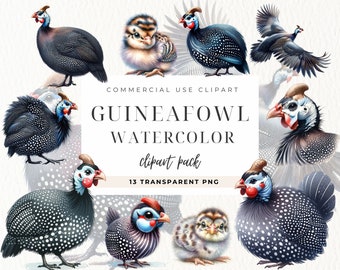The image appears to be a cover or thumbnail for a downloadable clip art pack. It features a slightly blurred, smaller-sized image with a central white rectangle containing text. At the top in small letters, it says "Commercial-Use Clipart." In the center, larger letters read "Guinea Fowl Watercolor," and below that, in smaller cursive script, it says "clipart pack," followed by "13 transparent PNG" in even smaller text. Surrounding this text box are ten watercolor-style drawings of guinea fowl in various stages of life, including baby chicks, juveniles, and adults. The birds are depicted in multiple styles, some highly detailed and realistic, while others are pastel or cutely drawn. There's also an image showing a bird in flight with wings spread, adding to the diversity in representation. The guinea fowl are characterized by their polka-dotted feathering, round bodies, short legs, blue faces, and distinctive red jowls. The overall layout of the birds forms a rectangle around the central text, creating a visually engaging and informative presentation of the clip art pack contents.